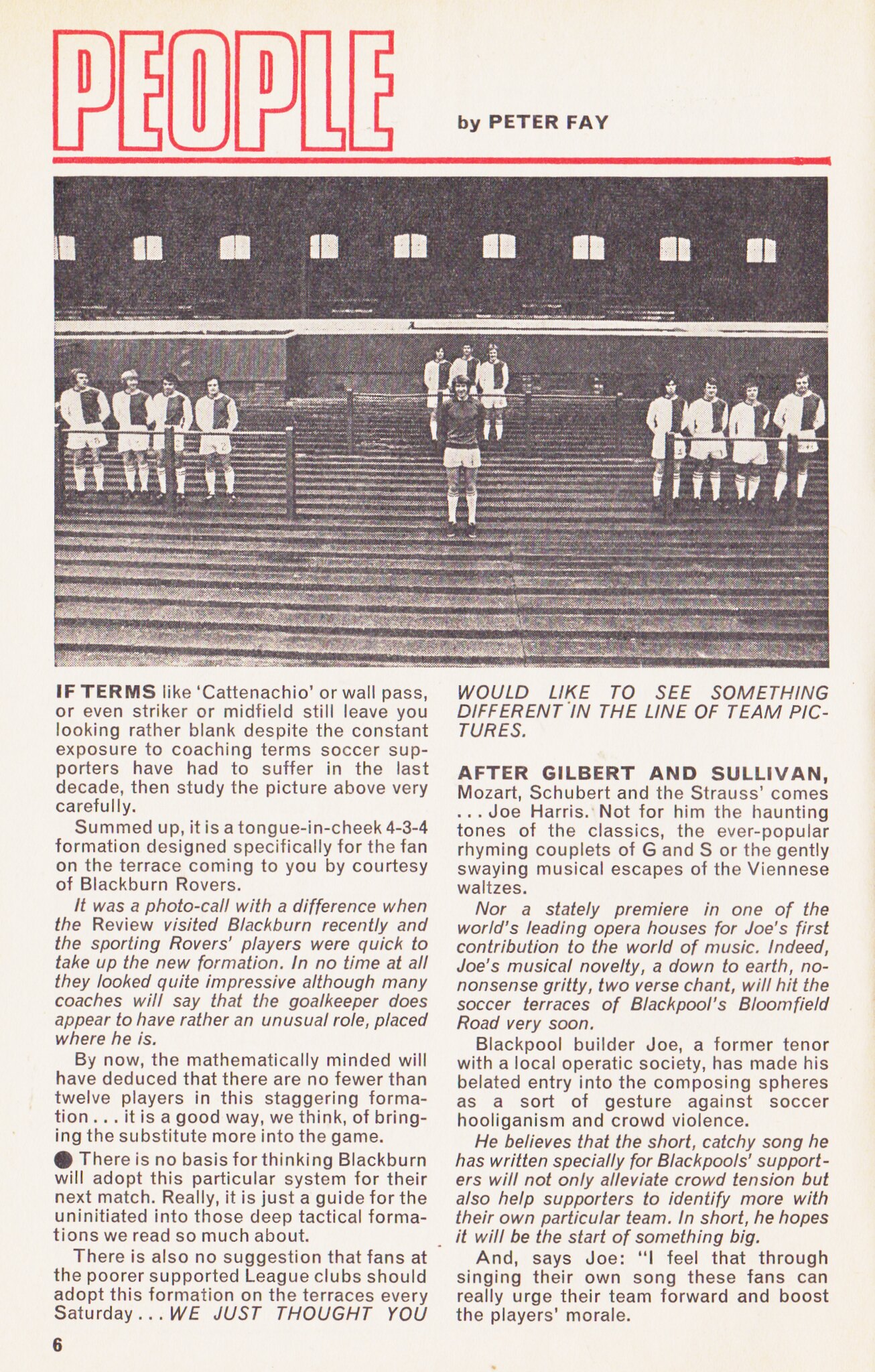The image is an excerpt from a magazine or newspaper, highlighted in the top left corner with "People" in bold red font, followed by "by Peter Fay" underlined. Below this heading, there is a photograph featuring a group of soccer players arranged in a 4-3-4 formation. This formation is described humorously as "tongue-in-cheek," intended for fans in the terraces. The players are dressed in a mix of uniforms, with one individual in the center donning a dark shirt, while others around him wear white shirts with dark accents. The caption beneath the photo reads: "Would you like to see something different in the line of team pictures?," indicating a novel approach to team photographs. The accompanying text jokes about soccer terminology like "casencio," "wall pass," "striker," and "midfield," suggesting that even with frequent exposure, many fans still find these terms confusing. The article credits Blackburn Rovers for bringing this creative team photo to the readers.